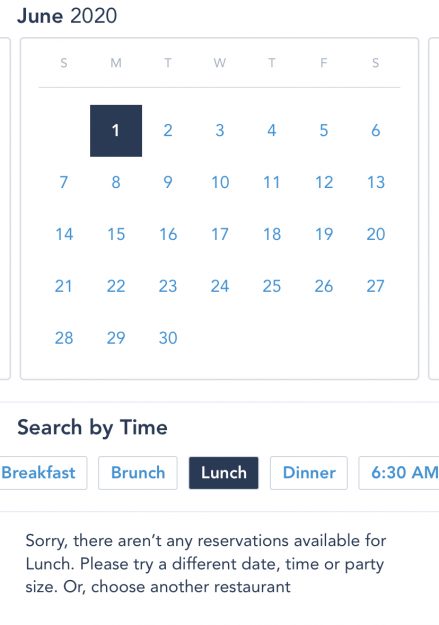This vertical rectangular image features a calendar view, presumably for booking a reservation. At the top, bold text reads "June 2020," followed by a smaller, thinly outlined gray box displaying the days of the week, abbreviated as S, M, T, W, T, F, S. Directly beneath this, the calendar days from 1 to 30 are presented. The first day of June falls on a Monday, highlighted with a blue box containing white numerals, while the rest of the dates are simply listed in blue text.

Below the calendar, there's a thin gray horizontal line. Larger text underneath reads "Search by Time." Following this, several rectangular options for different meal times are displayed: breakfast, brunch, lunch, and dinner, alongside a specific time slot labeled "6:30 AM." Each option is outlined with a thin gray border. The option for "lunch" is uniquely highlighted in a blue box with white text.

At the bottom of the image, a message indicates, "Sorry, there aren't any reservations available for lunch. Please try a different date, time, or party size, or choose another restaurant." The majority of the text in the image is presented in shades of blue, maintaining a cohesive color scheme.